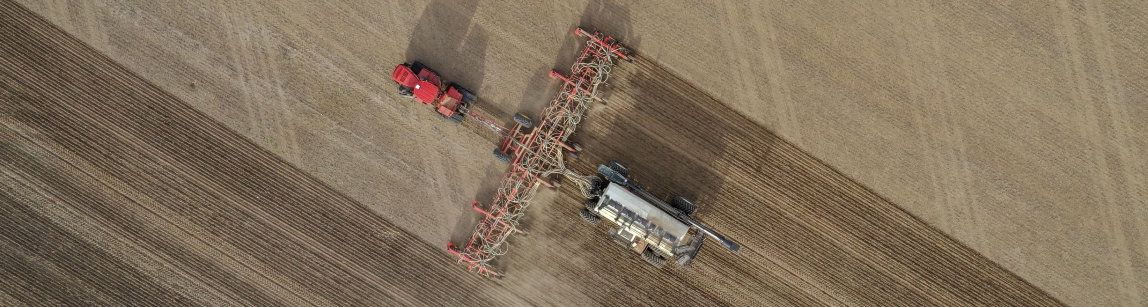This aerial photograph captures a moment on a farm where agricultural equipment is actively working the land. Central to the image is a red tractor moving diagonally towards the upper left corner, pulling behind it two distinct machines. The first machine, directly attached to the tractor, is red and appears to be constructed of tubes and wires, likely serving to churn and smooth the soil. The subsequent machine is a silver tank on wheels, possibly serving as a seeder, depositing seeds into the freshly plowed ground.

The field itself tells the story of the work being done: the area behind the tractor is a darker brown, indicative of freshly tilled soil, while the untouched sections of the field remain a lighter brown. The field exhibits a grid pattern etched into the earth by the machinery, showing the progress and method of the agricultural process. The right side of the photograph appears lighter, with a straw-like color, while the left side is darker where the soil has been treated.

Overall, this detailed image showcases not only the machinery in use but also the contrasting states of the field, highlighting the ongoing agricultural activity from a unique, overhead perspective.